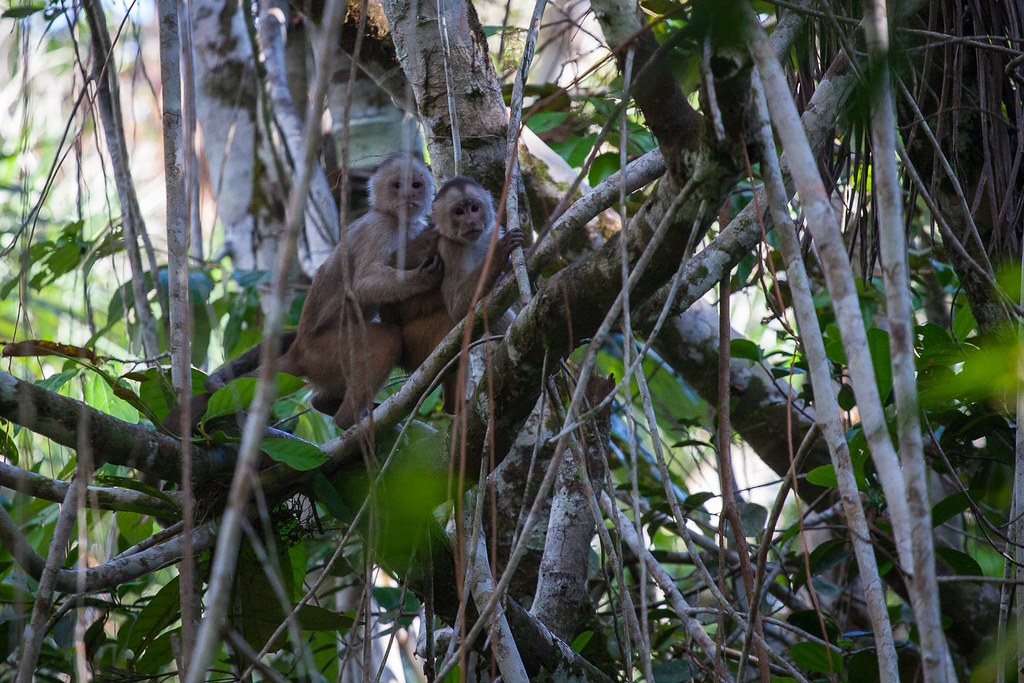In this photorealistic image, two small Capuchin monkeys are prominently featured nestled together in the midst of a lush, deciduous forest. They are perched on and clinging tightly to thin, pale white branches interspersed with green leaves. The monkeys, distinguishable by their black heads and white fur, appear almost human-like as one holds the other closely. While they remain mostly still, their inquisitive gaze is directed around their surroundings, dominated by light and dark brown trees. Some branches, appearing out of focus in the background, create a layered depth to the scene. The forest floor at the three o'clock side is carpeted with moss, and the sunlit ambiance suggests a bright, cheerful day. The overall setting brims with vibrant greenery, with potential hints of bamboo and large-leaved plants, evoking a serene and natural environment, possibly even a section within a zoo enclosure.